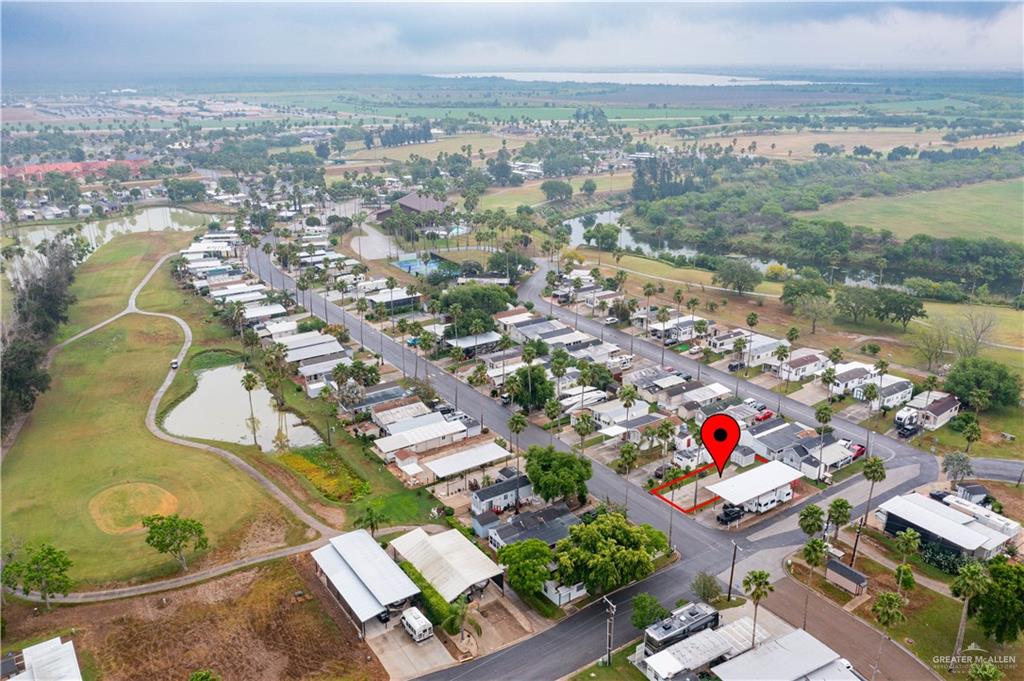The image depicts an overhead view of a small community consisting mainly of trailers and RVs, adjacent to a sprawling golf course with visible cement cart paths that form a fork and a loop. The community is characterized by numerous white and gray-roofed buildings, possibly businesses, and residential structures. A prominent red pinpoint marker highlights a specific, seemingly unoccupied building within the community. Surrounding the area are plentiful trees, a green field—part of which is likely the golf course—and a scattering of clouds. In the background, a field bordered by trees is noticeable, along with a row of houses and buildings, culminating in distant low hills. The scene also includes isolated elements like a small factory, further adding to the diverse landscape of the picture.